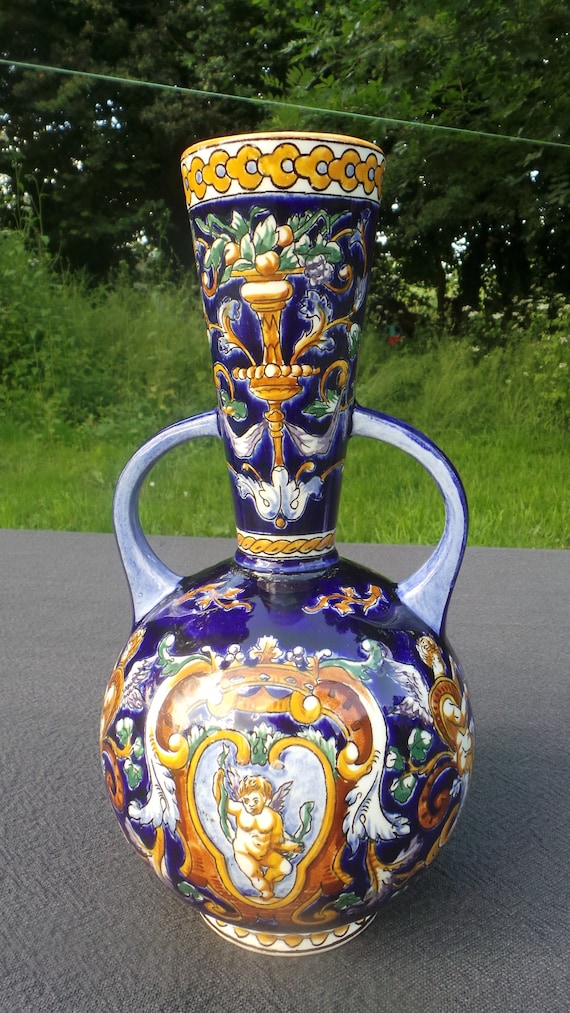The photograph showcases an intricate antique porcelain carafe, prominently positioned on a gray cement walkway. This carafe features a unique design with a narrow, conical neck and two light blue handles that connect to the bulbous, circular base. The primary color of the carafe is a rich dark blue, adorned with elaborate gold and green decorative elements. 

At the neck of the carafe, a striking gold emblem resembling a sword is prominently displayed, accented by golden apples and green leaves. Below this emblem, the vase transitions into a larger circular base, which is encircled by a detailed pattern of gold and green petals. Central to this lower portion is a depiction of a cherubic, winged baby, enclosed within a heart-shaped frame that gives off a golden hue. This figure, resembling a mythological character or angel, adds a touch of whimsy and intricacy to the overall design. 

The carafe sits amidst a natural setting, with lush green grass, taller weeds, and tree branches filled with verdant leaves visible in the background. The detailed craftsmanship and natural backdrop combine to create a striking and picturesque composition.